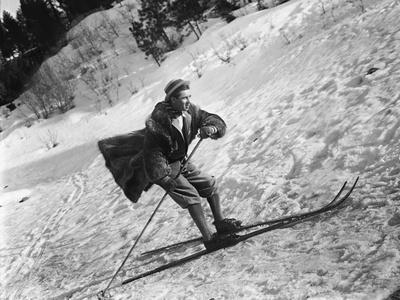This vintage black and white photograph captures a man engaging in an attempt to ski across a snowy, slightly slanted landscape that appears mostly flat. The skier, a Caucasian man with pale skin, is dressed somewhat inappropriately for freezing temperatures, wearing a thin, flowing fur coat and equally thin pants. His attire also includes a hat, which could be a top hat, adding an antique charm to his appearance. He holds a pole in his left hand, his arm bent at the elbow as he plants it into the snow to help propel himself forward. Despite the generally flat terrain, he is angled slightly to the top right and looks determined in his movements. The background features a snow-covered hillside with scattered trees, setting the scene beautifully. This photograph, likely taken in Lake Placid, New York, exemplifies vintage photographic representationalism with strong elements of realism.